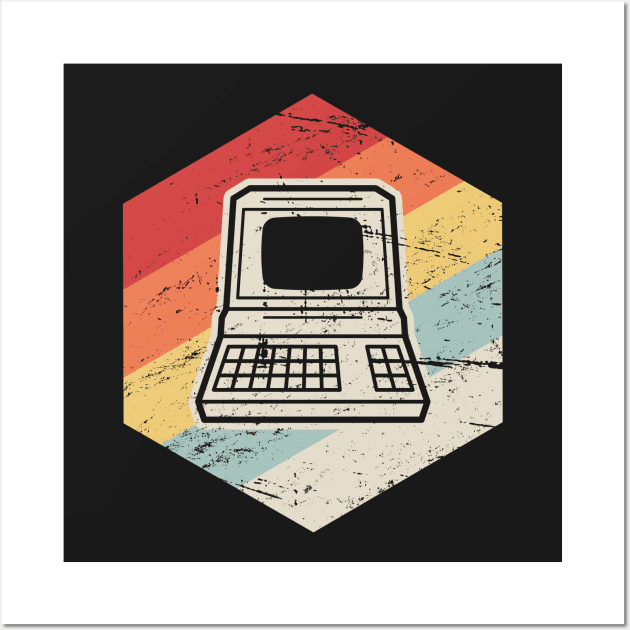This artwork features a centrally placed hexagonal geometric shape within a square frame, all set against a contrasting white border and dark black background. The hexagon is adorned with a vibrant gradient of lines that streak diagonally from the top left to the bottom right in a progression of colors: red, orange, yellow, light blue, and white. Within the center of the hexagon lies a meticulously detailed black-and-white sketch of a vintage cash register, complete with multiple buttons on its base and a prominent display screen. The overall composition juxtaposes the vivid and dynamic outer patterns with the intricate and monochromatic central figure, creating a striking visual balance.